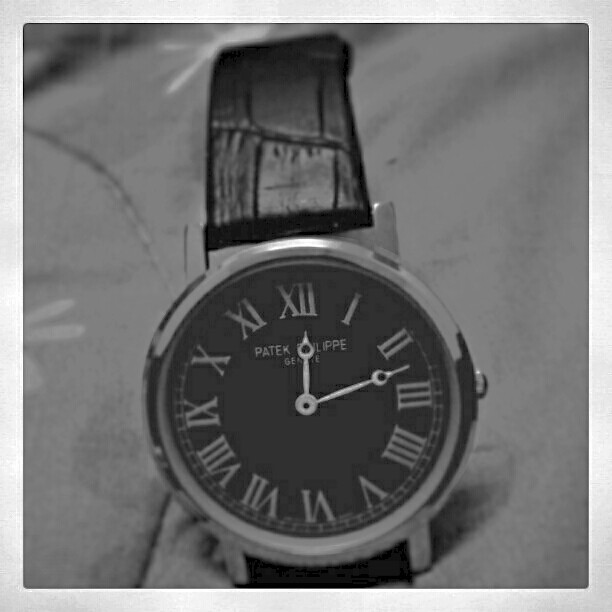The image features a luxurious wristwatch prominently placed on a textured grey surface, possibly a soft fabric like a blanket. The watch has a sleek, reflective silver body with a matching silver knob located on the right side. Its strap is black, potentially made of leather or faux leather, and is intricately designed with a pattern resembling scales or small rectangles and squares. The watch face is a striking black circle adorned with white Roman numerals: XII at the top, III on the right, VI at the bottom, and IX on the left, with all the intermediate numbers present. In the upper center of the watch face, beneath the XII, "Patek" is written in white, though additional text is partially obscured by the hands of the watch. The dials are slender and silver, with the shorter hand pointing at XII and the longer hand positioned between II and III. This digital photograph is framed with a white border, giving it a vintage Polaroid appearance.